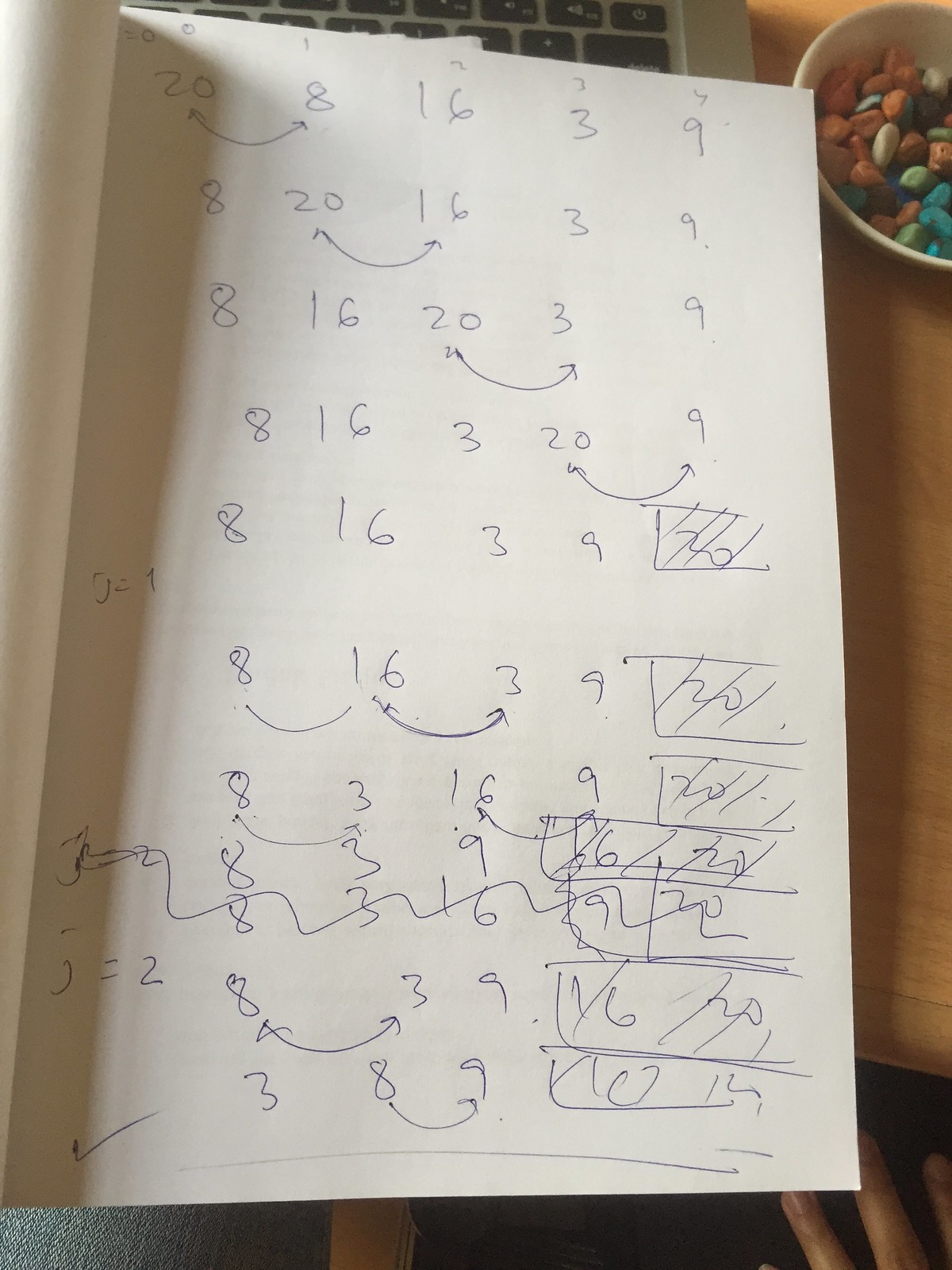A meticulously arranged workspace features an open notebook resting on a white, tan-wooden table. The notebook, positioned atop a keyboard, reveals a series of handwritten numbers on an unlined page. At the top of the page, the numbers are organized as follows: "20, 8, 16, 3, 9," with arrows connecting "20" to "8." The pattern continues in subsequent lines with variations in the numbers and connecting arrows, eventually leading to lines filled with scribbles and a checkmark at the bottom.

Adjacent to the notebook and keyboard, in the upper right corner of the image, sits a white bowl containing an assortment of snacks. The contents appear to include peanuts, blue and green snack pieces, and yogurt-covered raisins. Both the keyboard and the bowl of snacks partially intrude into the frame, adding context to the workspace's setting. The clean, organized layout emphasized by the bright, natural wood surface highlights a blend of productivity and leisure.